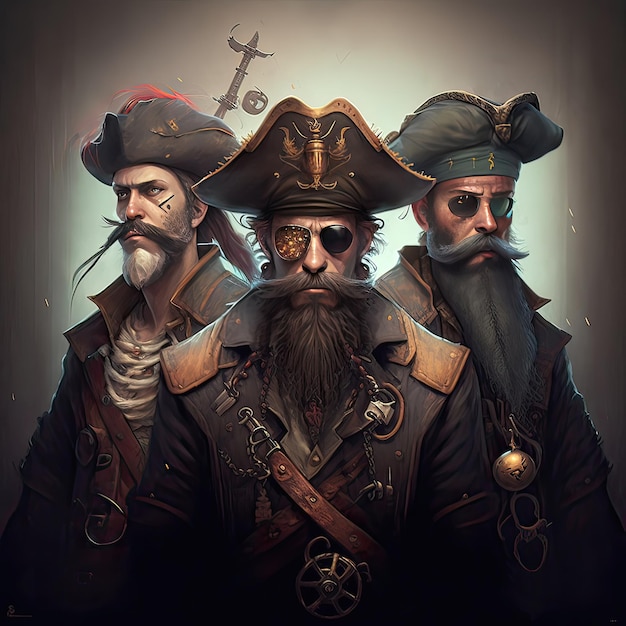The image depicts a detailed digital painting of three pirates in 17th-century attire, standing against a dark background with a white circle behind their heads. The central pirate, looking directly at the viewer, dons asymmetrical sunglasses, a twirled mustache, and a beard. His clothing includes a dark blue and black ensemble with leather shoulder pads, various gold chains, and a cross-body belt from his right shoulder to his left hip.

Flanking him are two other pirates; one gazes to the right and the other to the left. Each pirate sports a tricorne hat with gold trim and various accessories, including feathers and gold jewelry. Two of the pirates wear sunglasses while all feature long beards and thick mustaches. Their outfits are predominantly dark in color, with brown and gray elements, and are accented with gold details. The overall scene captures the rugged and opulent essence of pirate life in a striking and cohesive visual manner.